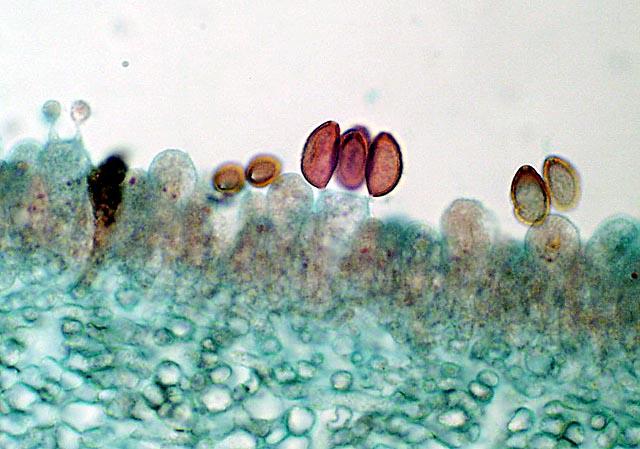The image depicts a highly magnified slide, likely viewed under a microscope, featuring a complex and textured array of elements. Dominating the majority of the image are myriad small, green dots that resemble scales, each displaying ridges that suggest a rough texture. These green dots sit against a watery, grayish background. Interspersed among them are a few distinct, red circular shapes—specifically, three red dots—that stand out due to their rarity and bright color. Additionally, the image showcases other multicolored, pumpkin seed-shaped objects in the center, ranging from plum, purpley-orange, and yellow to gray tones. These central objects, with their varied hues and outlined edges, give the impression of cells or shells. The visual composition of the painting or photograph includes a base of greenish-blue marbles that collectively create a dense foundation, while the top of the image is marked by a white background that contrasts the vivid colors below. Overall, the depiction of these tiny, diverse components conveys the sense of an electron microscope image, offering an intricate look at microscopic life forms or specimens.